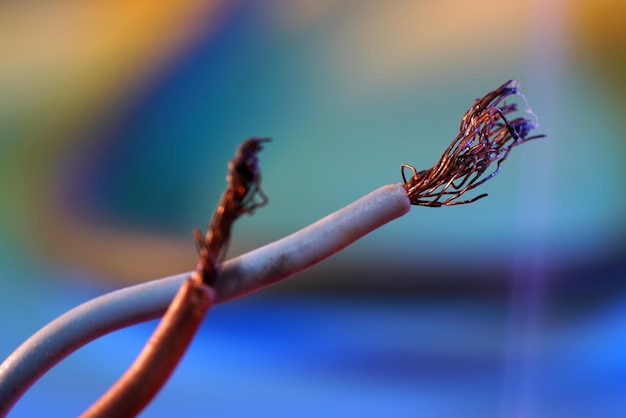In the photo, there are two wires with frayed ends, almost as if the rubber insulation has been cut away to expose the copper strands inside. The white wire, positioned in the background, appears shorter and crosses over the longer red wire in the foreground. The internal copper wires are thin and numerous, fanning out from the ends where the cuts are. The backdrop is notably blurry, featuring a predominantly blue hue with hints of green and occasional orange and yellow tones. The photo is clearly focused on the two frayed wires, highlighting the contrast between their exposed copper innards and the blurry, multicolored background.